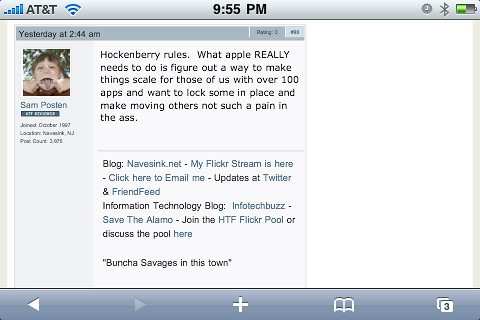This detailed screenshot captures a forum post by Sam Polston, as displayed on a phone screen with AT&T service. The phone shows typical interface elements such as the battery icon, signal bars, and the time, indicating a late night timestamp of 2:44 a.m. 

The forum post, highlighted under Sam Polston’s name, includes his profile picture of a child making a funny face into the camera. Sam, an old member of the forum with over 3,000 posts, wrote: "Hockenberry rules. What Apple really needs to do is figure out a way to make things scale for those of us with over 100 apps and want to lock some in place and make moving others not such a pain in the ass."

Following his message, there are clickable links to his blog, knavesync.net, and various contact points such as his Flickr stream, email, Twitter, and friend feed. The post rounds off with statements about participating in the information technology blog community and a mention of joining the HTF Flickr pool or discussing it. At the very bottom, a casual remark reads, "bunch of savages in this town."